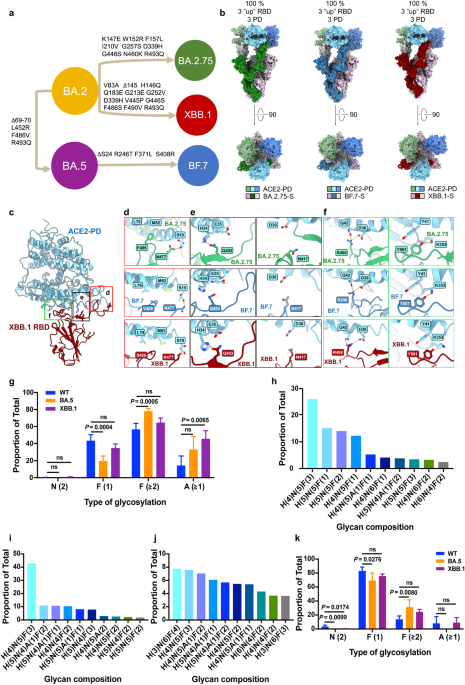This image showcases a detailed scientific diagram likely from a manual or technical document. At the top, there are colorful plant-like illustrations with labels indicating different percentages and conditions, such as "100%," "3PD," and "AC something PD." Below these illustrations, there are five bar charts. These charts feature data on different types of glycosylation. Each bar graph is color-coded with shades of blue, purple, green, orange, red, turquoise, and yellow. The vertical axes on these charts are labeled with terms like "proportion of total" and "HC glycan composition." 

Interspersed among the charts are small colorful circles, each containing white text, with labels like "BA2," "BA5," "F7," "XBB1," and "BA2.75." These circles are connected by arrows pointing to associated data points, although the text is too small to decipher clearly. The diagram also includes an area labeled 'C' that resembles a map, filled with squares outlined in various colors such as red, blue, and green, each containing additional data. The complexity and variety of visual elements suggest a multi-layered presentation of scientific data, rich in graphical and numerical information.